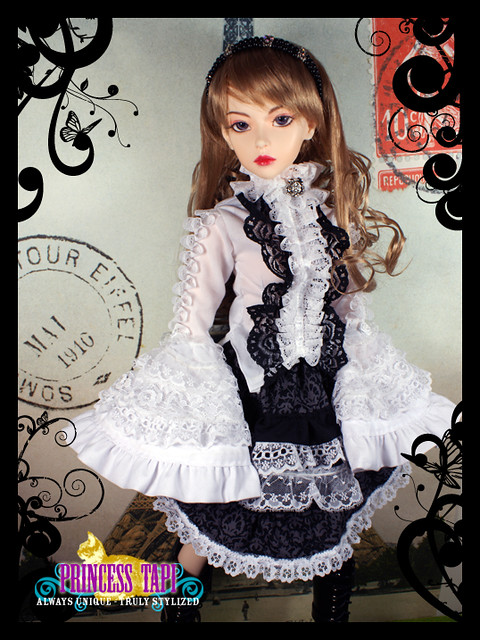The image is a detailed photograph resembling a collectible French-made doll or possibly the cover of its packaging. Framed by a quarter-inch black border, the image measures about four inches wide by six inches long. In the center of the image stands a porcelain doll with wavy, strawberry-blonde hair cascading over her shoulders. Her skin is white, and she features distinct brown eyebrows, large widely-set eyes, a small nose, and lips outlined in soft red lipstick, giving her a dainty, almost lifelike appearance.

The doll is dressed in a delicate, frilly outfit that seems reminiscent of a French maid or cocktail waitress costume. She wears a long-sleeved white blouse with bell-shaped cuffs that extend beyond her hands, adorned with layers of lace. Over the blouse, she dons a black apron with black lace detailing and numerous layers of white lace both around the neck and down the front. Her short skirt features additional layers of lace at the bottom, completing the detailed attire. She also wears small black boots, with a glimpse of her ankles visible.

In the lower left-hand corner of the image, the doll's name, "Princess Tari," is written in large purple capital letters. Below this, in small white capital letters, is the phrase, "always unique, truly stylized." The background features intricate black patterns and curlicue designs, with hints of a golden cat image partly obscured by the text. Additionally, there is a partially visible postage stamp on the left side, bearing the date May 1910, suggesting historical or collectible significance.

In the upper right corner, a red sticker with the number "10" printed on it adds to the visual complexity of the image, enhancing its vintage appeal. The overall composition, decorative elements, and historical references make this photograph a captivating depiction of a meticulously crafted doll.